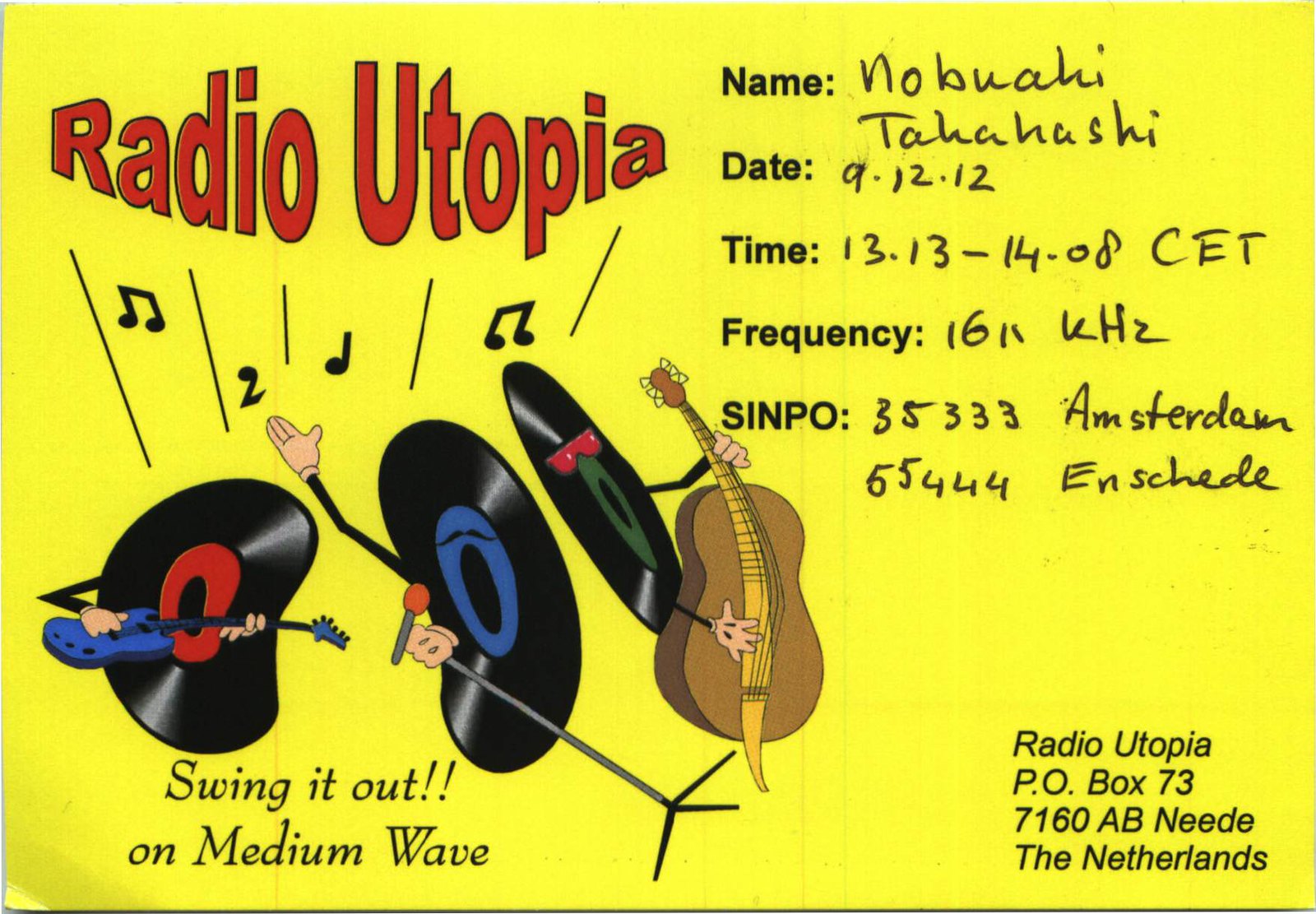The image depicts a vibrant, cartoonish poster with a yellow background, titled "Radio Utopia" in red text located in the upper left corner. The main illustration features three animated vinyl records: one playing a blue guitar, another singing into a red microphone, and the third playing a brown floor-standing bass. These records are black, red, and blue, with expressive mouths adding to their lively, musical performance. Below this whimsical trio, the black text reads "Swing It Out on Medium Wave." In the upper right quadrant, detailed event information is provided: Name – No Booty Takahashi; Date – 9-12-12; Time – 13:13-14:00 CET; Frequency – 16 kHz; and Signal Reception reports as SINPO (Signal, Interference, Noise, Propagation, Overall) 35333 for Amsterdam and 55444 for Enschede. The poster also features musical notes throughout, accentuating its thematic focus on music. In the lower right corner, the address for Radio Utopia is listed as P.O. Box 73, 7160 AB Neede, The Netherlands.